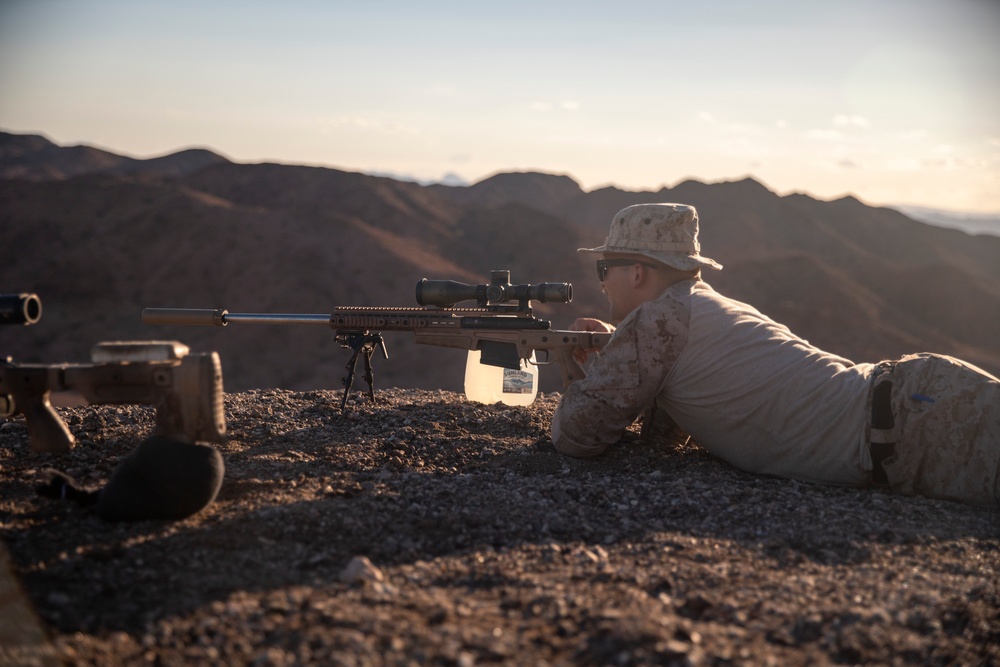The photograph captures a man who appears to be a military sniper, lying prone on a surface covered in small pebbles and dirt. Clad in a beige desert camouflage outfit, including a sun hat, camouflage-slippery sleeves on a grayish-tan shirt, and matching camouflage pants, the man intently looks through the scope of a long-range sniper rifle, which is supported by a bipod. His face is partially obscured by sunglasses. Nearby, there is a milk jug filled with water situated to his right and another propped-up rifle to his left, although it's unclear if this second rifle belongs to him or someone else. The background features a picturesque view of distant mountains under a sky that transitions from a mild orange at the horizon to a blue-gray higher up, suggesting either early morning or late evening.